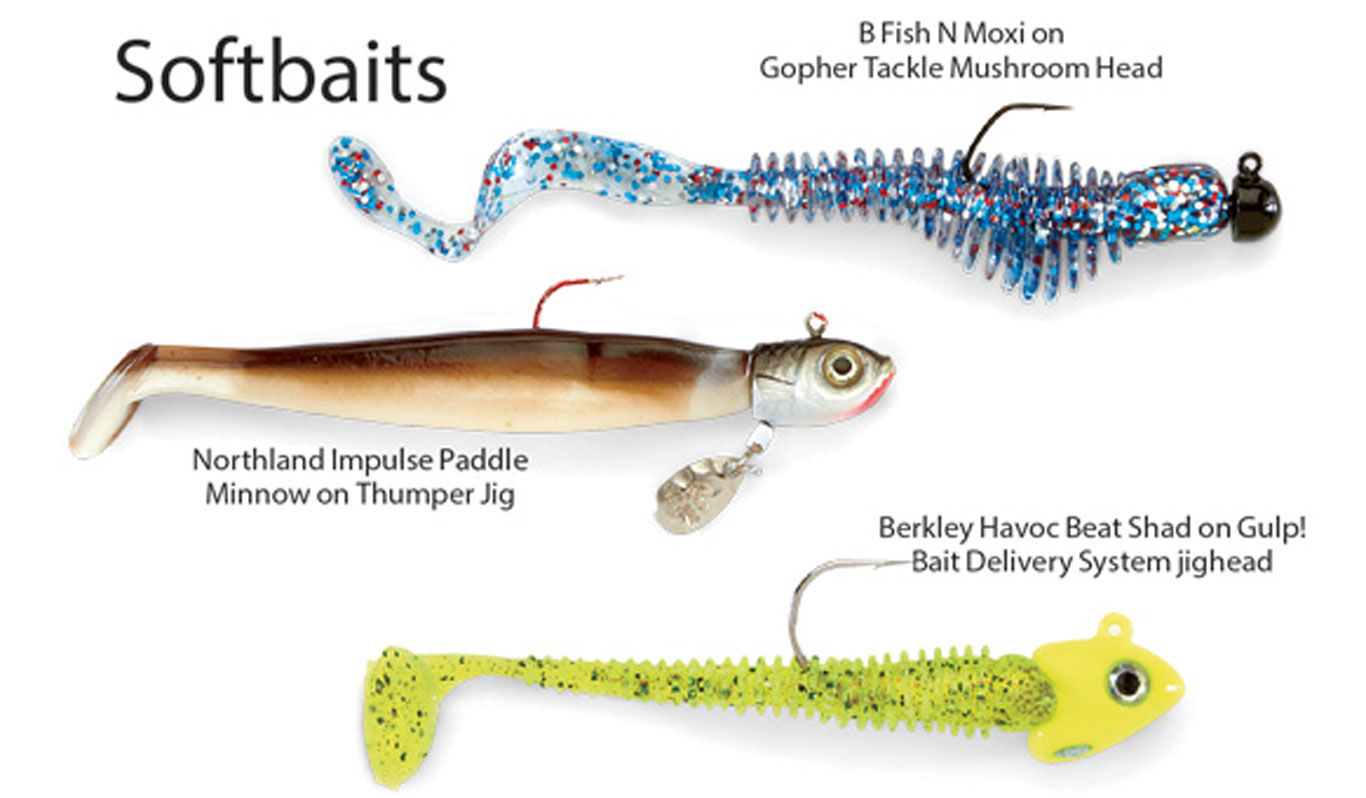This is a detailed photograph of various soft baits used for fishing, each labeled with specific tackle information. At the top, a glittery lure named "Beefish M. moxie on Gopher Tackle Mushroom Head" shines with blue, red, and white sparkles. It features a black head with a hook emerging from its back. The middle lure is a "Northland Impulse Paddle Minnow on Thumper Jig," characterized by a silver head and an eye, with a realistic brown body and another hook extending from its back. At the bottom, the "Berkley Havoc Bait Shad on Gulp! Bait Delivery System Jighead" stands out with its bright yellow head and greenish-yellow body speckled with glitter, along with a hook protruding from its spine. All three lures are soft and squishy, designed in worm-like shapes, perfect for attracting fish. The image prominently displays the phrase "Soft Baits" to emphasize the type of fishing tackle being showcased.